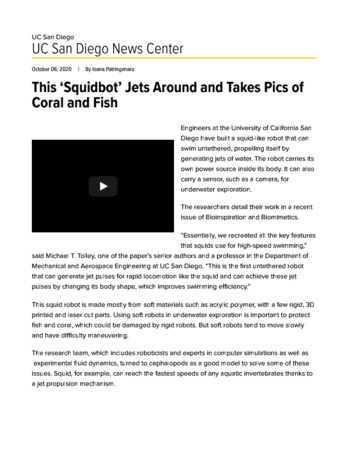This image appears to be a screenshot of an article from the UC San Diego News Center, dated October 6th, 2020. The article highlights a breakthrough by engineers at the University of California San Diego, who have developed a squid-like robot capable of swimming untethered. This innovative robot propels itself by generating jets of water and can carry its own power source within its body. Furthermore, the robot is equipped to carry sensors, such as a camera, making it suitable for underwater exploration by capturing images of coral and fish. The screenshot also features a black box with a white play button indicating the presence of a clickable video link in the original article. The author's name is not clearly visible.